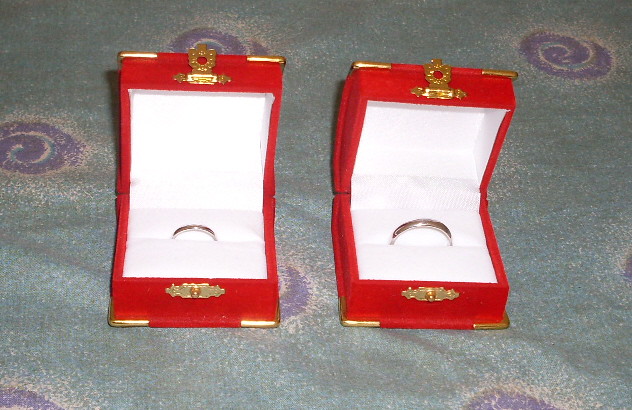In this photograph, two identical, bright red ring boxes are showcased side by side, both with open lids revealing white interior linings that appear to be made of a satiny velvet material. Each box features elegant gold accents, including gold trim and a delicate gold clasp at the top, which latches onto a matching gold knob at the bottom when closed. Inside, one of the boxes holds a small silver band that appears to be for a female, while the other contains a slightly larger silver band, likely for a male, suggesting they are matching wedding bands.

The boxes are displayed on a piece of material with a bluish-green hue, adorned with purplish swirl patterns. The fabric seems aged and slightly faded, with the color transitioning to a light gray or brown around the swirls. The photograph is taken from a slightly high, angled side perspective, with no text or people present in the image, allowing full focus on the elegant presentation of the ring boxes and their contents.